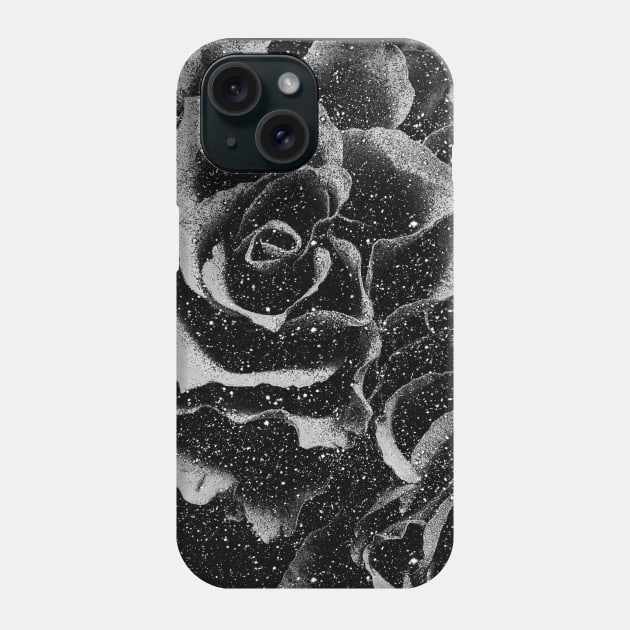This photograph showcases an iPhone, possibly an older model, placed on a plain grey background. The case adorns a detailed black-and-white depiction of multiple roses with curvy petals, giving it an abstract yet beautiful appearance. Scattered across the case are numerous white dots, reminiscent of either water droplets or decorative paint splashes, adding a romantic and intricate touch. The iPhone features two diagonally-aligned camera lenses and a flash, indicative of its advanced functionality. The phone has rounded corners, implying a sleek design. The case itself appears to be more rigid rather than soft, highlighting its stylish and protective features.